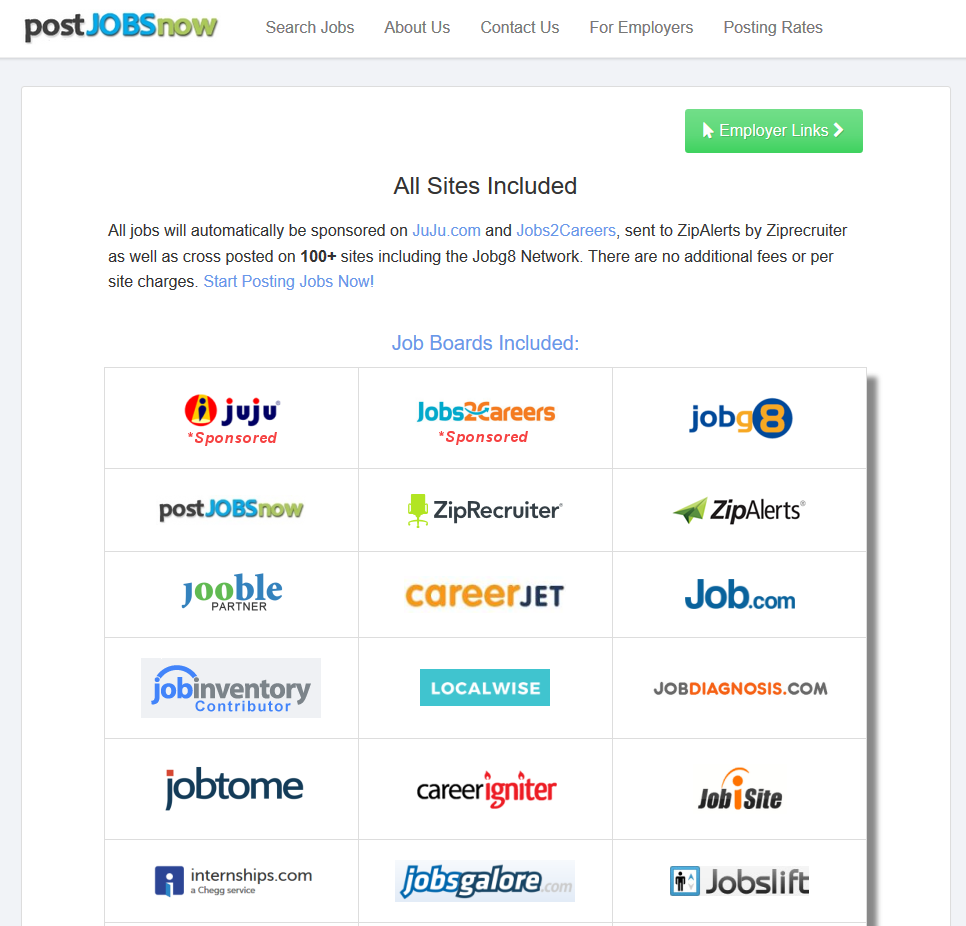In the image, various elements are laid out in an organized grid format. 

On the top left corner, the words "Post" are displayed in black text, "JOBS" in uppercase blue text, and "now" in lowercase green text. To the right, a green rectangle features the text "Employer Links." Beneath it, "All sites included" is written in black, and "Job boards included" appears in blue.

The grid comprises multiple rows, each with three sections:

1. The first row features:
   - "Juju Sponsored" in the first square.
   - "Jobs to Careers," where "Jobs" is in blue and "to Careers" in orange, in the second square.
   - "Job G8" in the third square.

2. The second row features:
   - "Post Jobs Now" in the first square.
   - "ZipRecruiter" in the second square.
   - "Zip Alerts" in the third square.

3. The third row features:
   - "Jubil Partner" in the first square.
   - "Career Jet" in the second square.
   - "Job.com" in the third square.

4. The fourth row features:
   - "Job Inventory Contributor" in the first square.
   - "LocalWise" within a blue rectangle in the second square.
   - "JobsDiagnosis.com" in the third square.

5. The fifth row features:
   - "JobTome" in the first square.
   - "Career Igniter" in the second square.
   - "JobSite" in the third square.

6. The final row features:
   - "Internships.com" in the first square.
   - "Jobs Galore" in bubble letters in the second square.
   - "JobsLift" in the third square.

Each section is neatly arranged and color-coded, creating a comprehensive and visually structured layout.